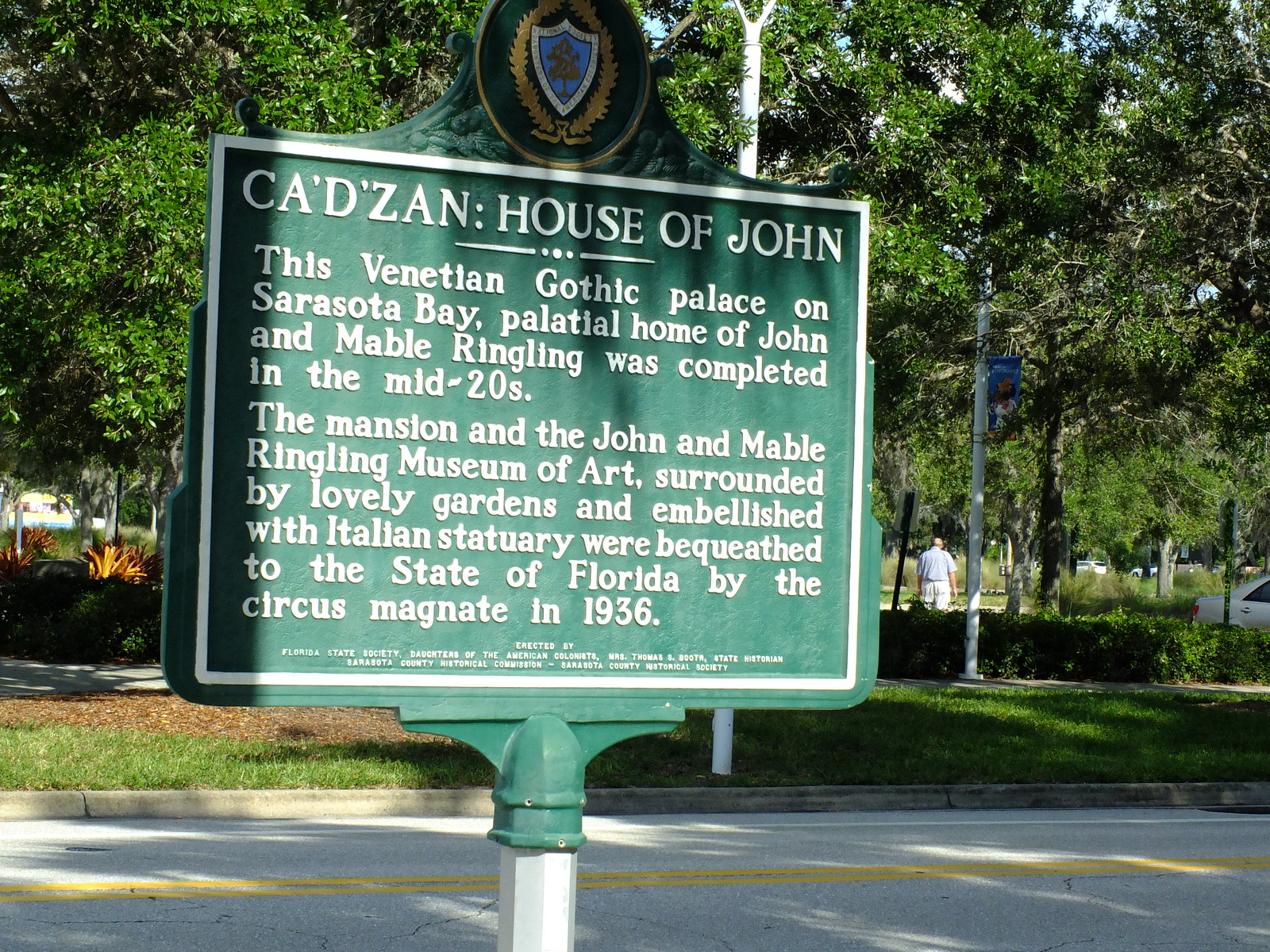The photograph captures an informational placard set in what appears to be a scenic park with manicured lawns, numerous trees, and a sidewalk. The sign is mounted on a sleek silver metal pole and is prominently green with a white border. At the rounded top of the sign, there's an intricate crest and shield logo that features a tree. The text on the sign is white and reads: "Kadzan, House of John. This Venetian Gothic palace on Sarasota Bay, palatial home of John and Mabel Ringling, was completed in the mid-twenties. The mansion and the John and Mabel Ringling Museum of Art, surrounded by lovely gardens embellished with Italian statuary, were bequeathed to the state of Florida by the Circus Magnate in 1936." The background of the image reveals a picturesque park with trees casting shadows on a small paved street marked by yellow double lines and extending from the bottom left to the bottom right of the frame. A person can be seen walking along a sidewalk, with lampposts and a partially cropped car visible in the scene.